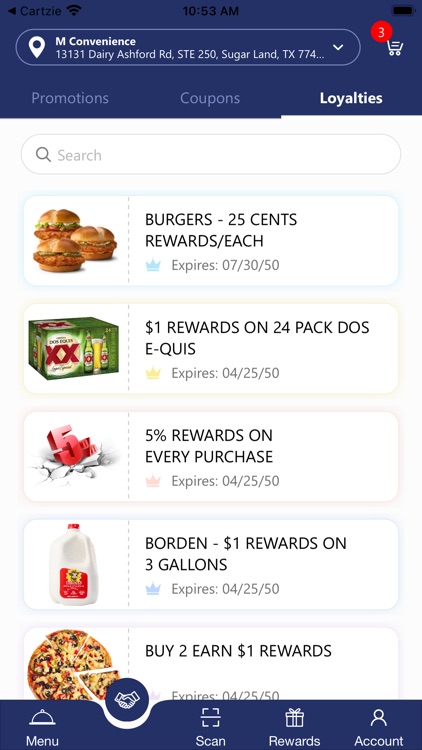This vertical image, captured from a smartphone, vividly displays a shopping app interface. At the very top, a blue rectangular bar houses several essential elements: the word "Cart" followed by the letter "C" in black at the upper left, a black Wi-Fi symbol, the time "10:53 a.m." in black text, and a battery life icon on the upper right.

Directly below this bar, a thin section labeled "M Convenience," along with an address on Derry Ashford Road in Sugar Land, Texas, features a circular shopping cart icon with the number "3" inside.

The main interface showcases promotions, coupons, and loyalty highlights against a light gray background. Dominating the center is a white search bar with a magnifying glass icon for easy navigation.

Below the search bar, the app presents various promotional offers, each accompanied by an icon:
- A burger icon labeled "Burgers," offering 25 cents rewards each, denoted by a small crown icon, with an expiration date of 7/30/50.
- A Dos Equis beer promotion, offering $1 rewards on a 24 pack, expiring on 4/25/50.
- A 5% rewards offer on every purchase, also expiring on 4/25/50.
- A gallon of Borden’s milk, offering $1 rewards on three gallons, with the same expiration date.
- A pizza icon indicating a "Buy two, earn $1 rewards" offer, expiring on 4/25/50.

At the bottom of the image, there are buttons labeled "Menu," "Scan," "Rewards," and "Account." Adjacent to the pizza icon, there's a smaller symbol depicting two hands shaking inside a circle, likely signifying a partnership or loyalty program.